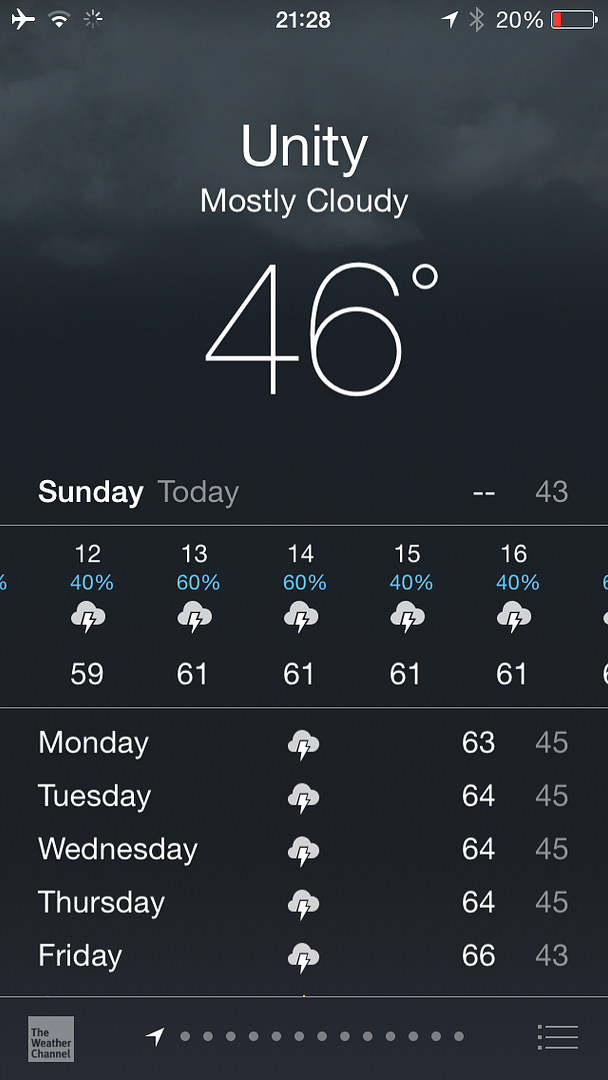The image depicts a screenshot of a smartphone display, highlighting various status and notification icons at the top of the screen. The phone is in flight mode, indicated by the flight mode icon on the top left, followed by the Wi-Fi icon and a searching/refresh icon, represented by a circular arrow. 

In the center of the top bar, the time is displayed as 10:28 AM. Adjacent to the time, additional icons include a live location icon and a Bluetooth icon. The battery percentage is critically low at 20%, indicated by the battery icon with a red line.

The background of the display shows a cloudy theme. Below the status bar, it reads "Unity, Mostly Cloudy, 46°F, Sunday, Today" with a double dash beside it, followed by the current temperature of 43°F. 

A sequence of numbers from 12 to 16 is displayed underneath, likely representing hours. Under each hour, respective percentages are shown: 12 (40%), 13 (60%), 14 (60%), 15 (40%), and 16 (40%), possibly indicating forecasted weather conditions or battery usage. Icons next to these times show a cloud with a lightning bolt.

Further down, there are day labels for the week: Monday, Tuesday, Wednesday, Thursday, and Friday, each accompanied by corresponding weather icons and numerical values on the left.